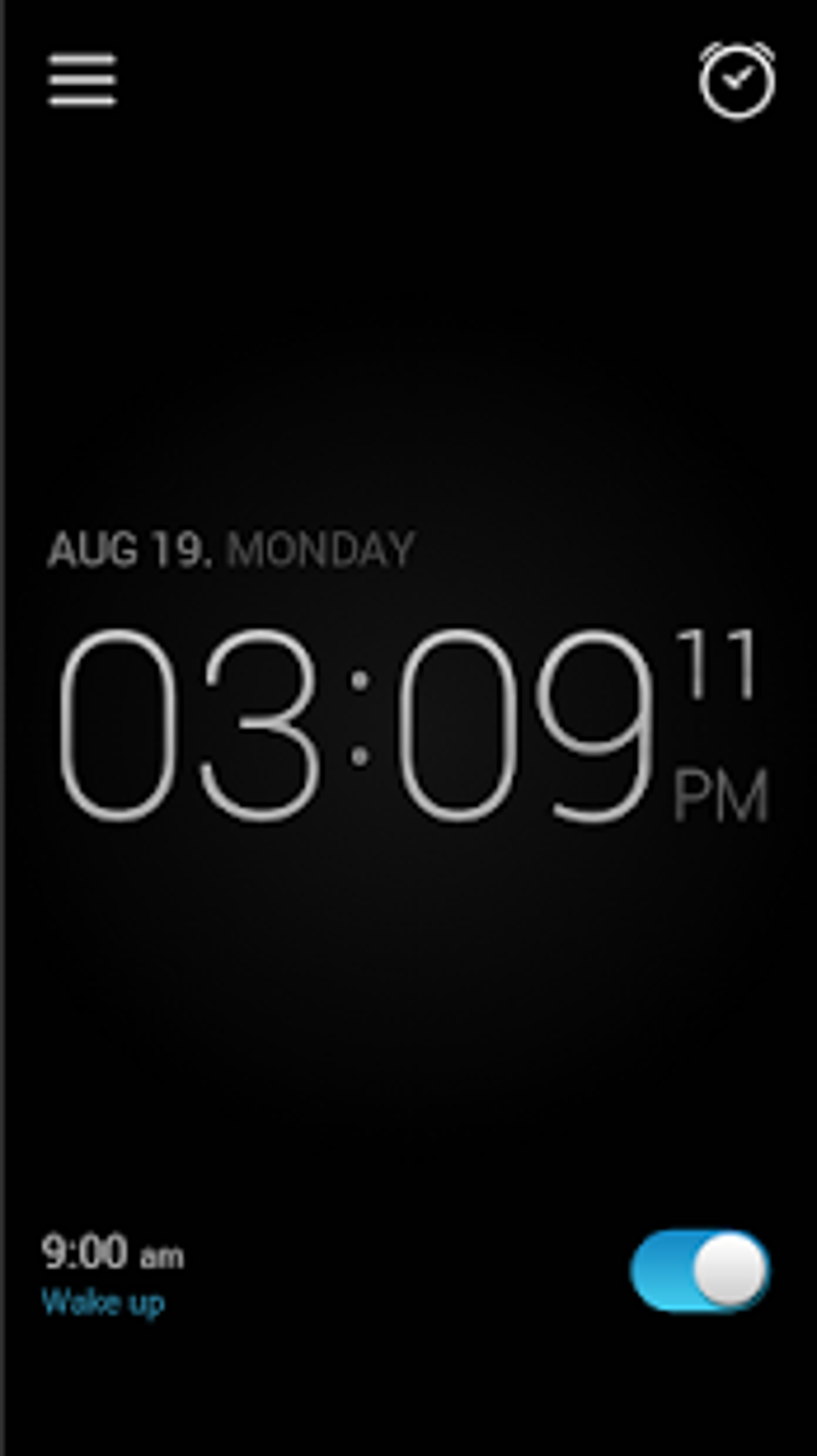This screenshot captures a mobile app designed as an alarm clock with a sleek, black background. At the top right corner of the screen, there's a small alarm clock icon, while the top left corner features a menu icon represented by three horizontal lines. In the center of the screenshot, the current time is prominently displayed in large white text, reading "3:09 PM." Positioned slightly above the "9," the number "11" appears, adding a distinctive detail to the time display. Directly above the time, a text reads "August 19 Monday," indicating the current date.

There is a significant blank space occupying the area between the top display and the bottom of the screen. At the bottom left corner, the time "9:00 AM" is indicated in smaller text, beside which is a label that reads "Wake up" with a blue underline. This indicates an active alarm that has been toggled on. The toggle button for this alarm is located to the right of this text and is highlighted in teal, signifying its active status. The overall design is minimalistic, drawing attention to the essential elements of time, date, and alarm settings against a completely black background.